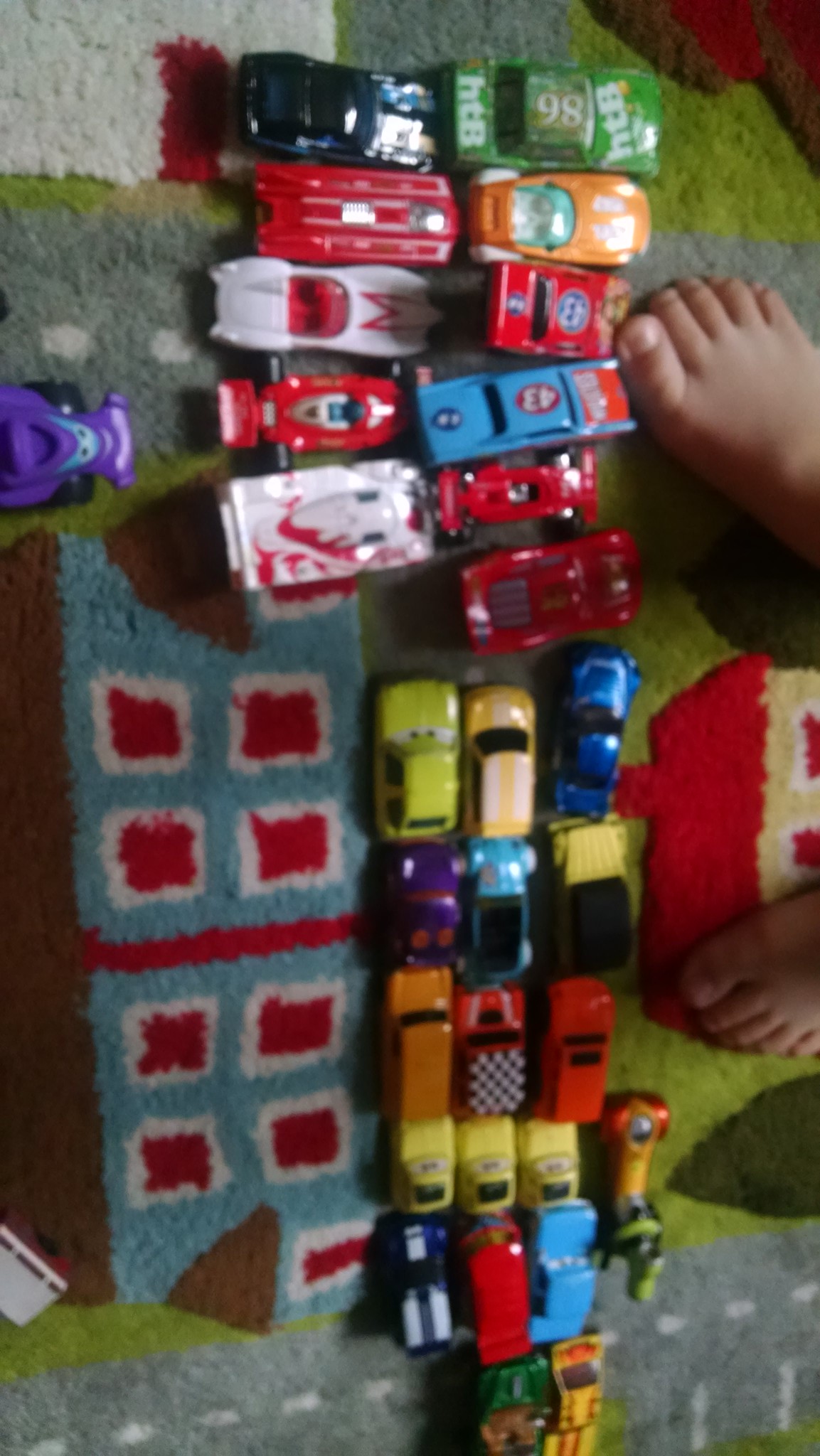The image showcases a colorful children's carpet featuring a detailed design, including a small house and a roadway. Positioned near the right-hand side of the image are the small bare feet of a child, which appear to belong to a young child. The carpet is covered with an array of toy cars, predominantly Hot Wheels or Matchbox cars, which seem to be meticulously arranged as if in a parking lot. The cars range in color and design, including a notable green car with "HTB" and "98" written in white, several VW Bugs, and cars with varying color patterns such as blue with white edges, a red car with white spots, and a white car with an 'M' marking on the front. There are approximately 28 to 30 toy cars, displaying a rich variety of colors such as blue, red, green, yellow, purple, black, and white. The cars stretch from the bottom to near the top of the carpet, predominantly centered, with some positioned along the left side. The intricate setup and vibrant detail illustrate a playful scene under the watchful presence of a young child.